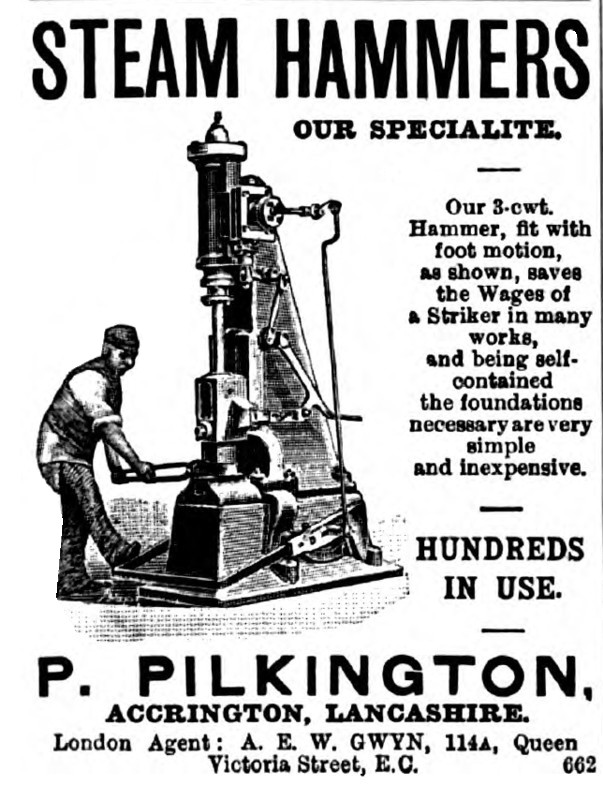This black-and-white image, seemingly from an old magazine advertisement, showcases a large industrial steam hammer from the late 19th or early 20th century. Dominating the left-hand side of the image, the machine features a prominent piston and a substantial hammer head, supported by a structure resembling a half-triangle. Below the hammer, a man operates foot motion pedals, enabling the mechanized process of metalworking, likely during the industrial age. The text wrapping around the image highlights the unique advantages of this steam hammer, emphasizing the cost-saving benefits of its self-contained design which requires minimal, inexpensive foundations. The advertisement proudly states: "Steam Hammers, Our Specialty. Our Three CWB hammer, fit with foot motion as shown, saves the wages of a striker in many works. Hundreds in use." Manufactured by P. Pilkington from Accrington, Lancashire, with a London agent AEW located at 1148 Queen Victoria Street, this steam hammer represents a significant advancement in industrial automation and efficiency.